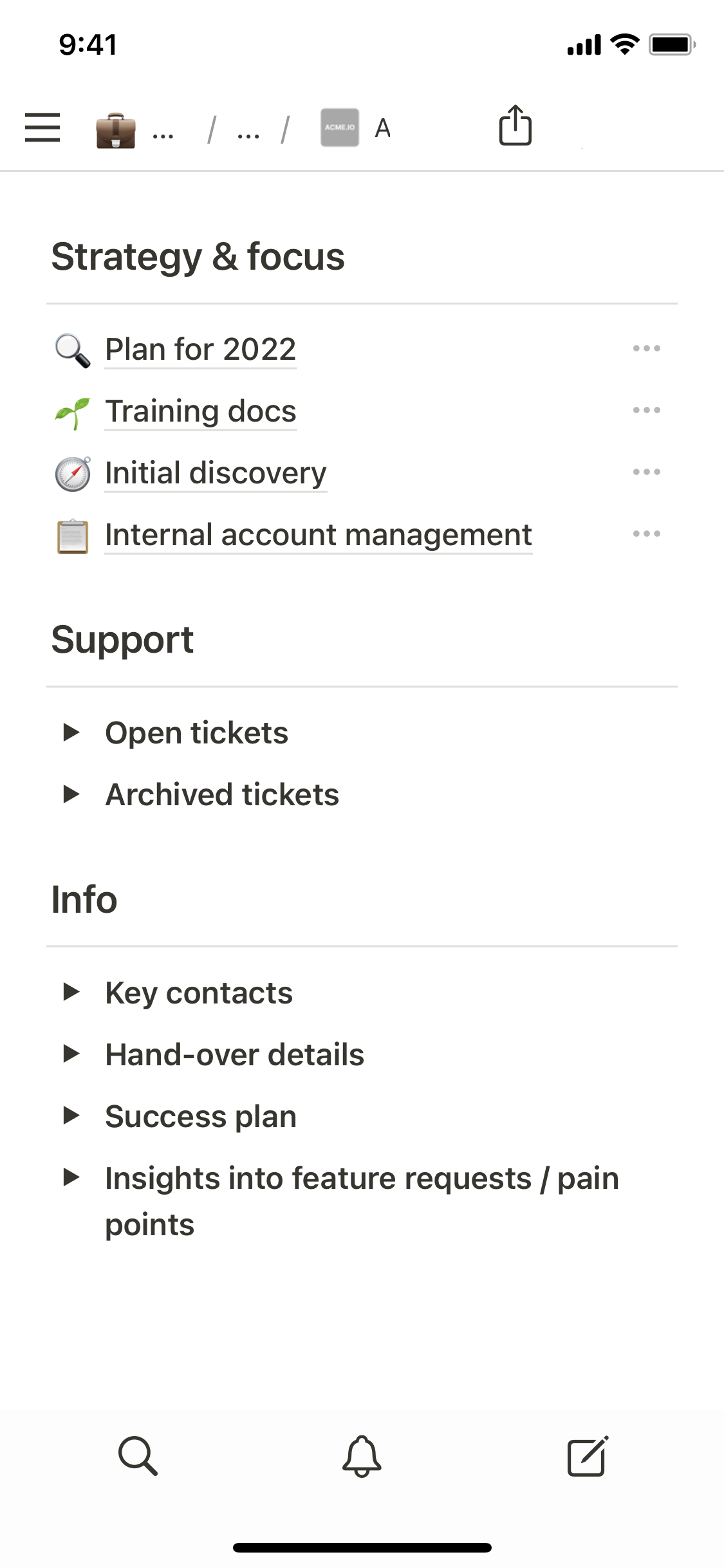The image is a detailed screenshot of a TAMON device interface. In the top left corner, the device model is indicated as TAMON 941. On the top right, the network signal strength is displayed with a full 4 out of 4 bars, Wi-Fi signal strength is shown as 3 out of 3 bars, and the battery indicator is present. 

The main body of the screen is organized into a series of text sections, covering various strategic and operational elements: 
- "Strategy and Focus"
- "Plan for 2022"
- "Training Docs"
- "Initial Discovery"
- "Internal Account Management"
- "Support"
- "Open Tickets"
- "Archive Tickets"
- "Info"
- "Key Contacts"
- "Handover Details"
- "Success Plan"
- "Insights into Future Requests"
- "Endpoints"

At the bottom of the screen are functional elements, including a search bar, a notification bar, and an edit bar.